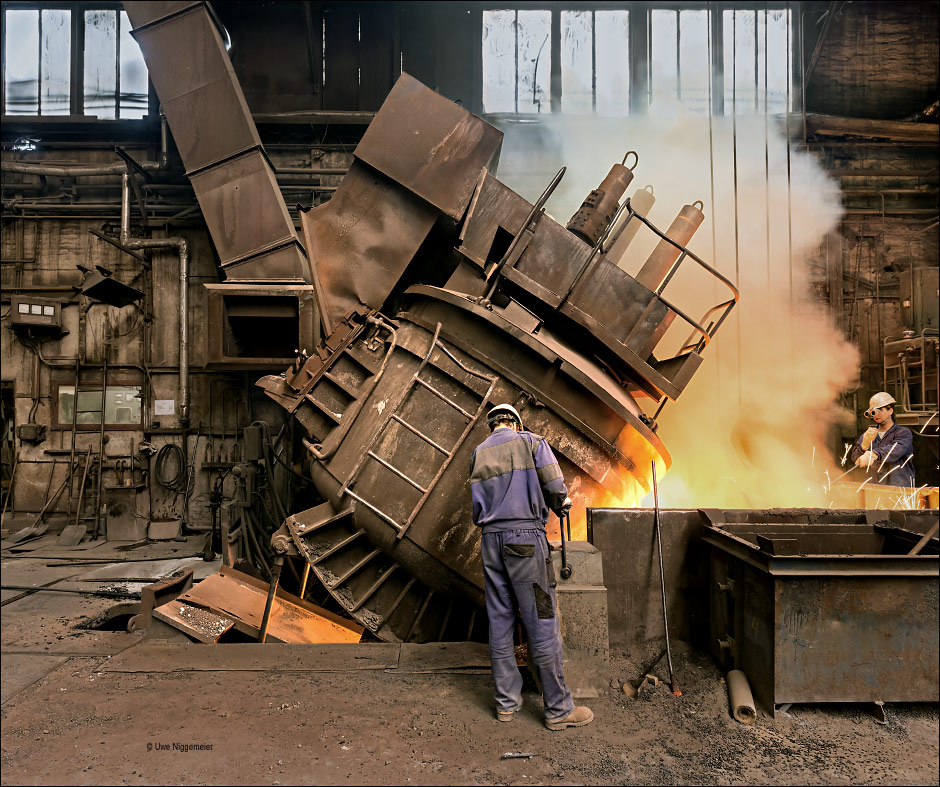The photograph captures a bustling and somewhat perilous scene inside an aged steel mill or foundry. The environment is rugged, featuring dirt floors and old wooden walls dotted with weathered windows. A significant presence in the image is a large, malfunctioning metal machine that is precariously tilting to the right, partially engulfed in fire and emitting heavy smoke. In the foreground, there are two men clad in blue work uniforms with white hard hats and steel-toe boots. The first man stands near the center, grasping a lever attached to a tall, rectangular vertical box, while the second man is positioned to the right, engaging with the molten metal in a glowing orange pool using a metal stick. Both men are enveloped in their work, under a grimy backdrop of tools, such as shovels, pipes lining the walls, and visible ductwork and electrical wiring. The overall vibe is one of intense industrial activity, filled with a sense of urgency and danger, highlighted by the vivid flames, billowing smoke, and general clutter that characterizes an active refinery.